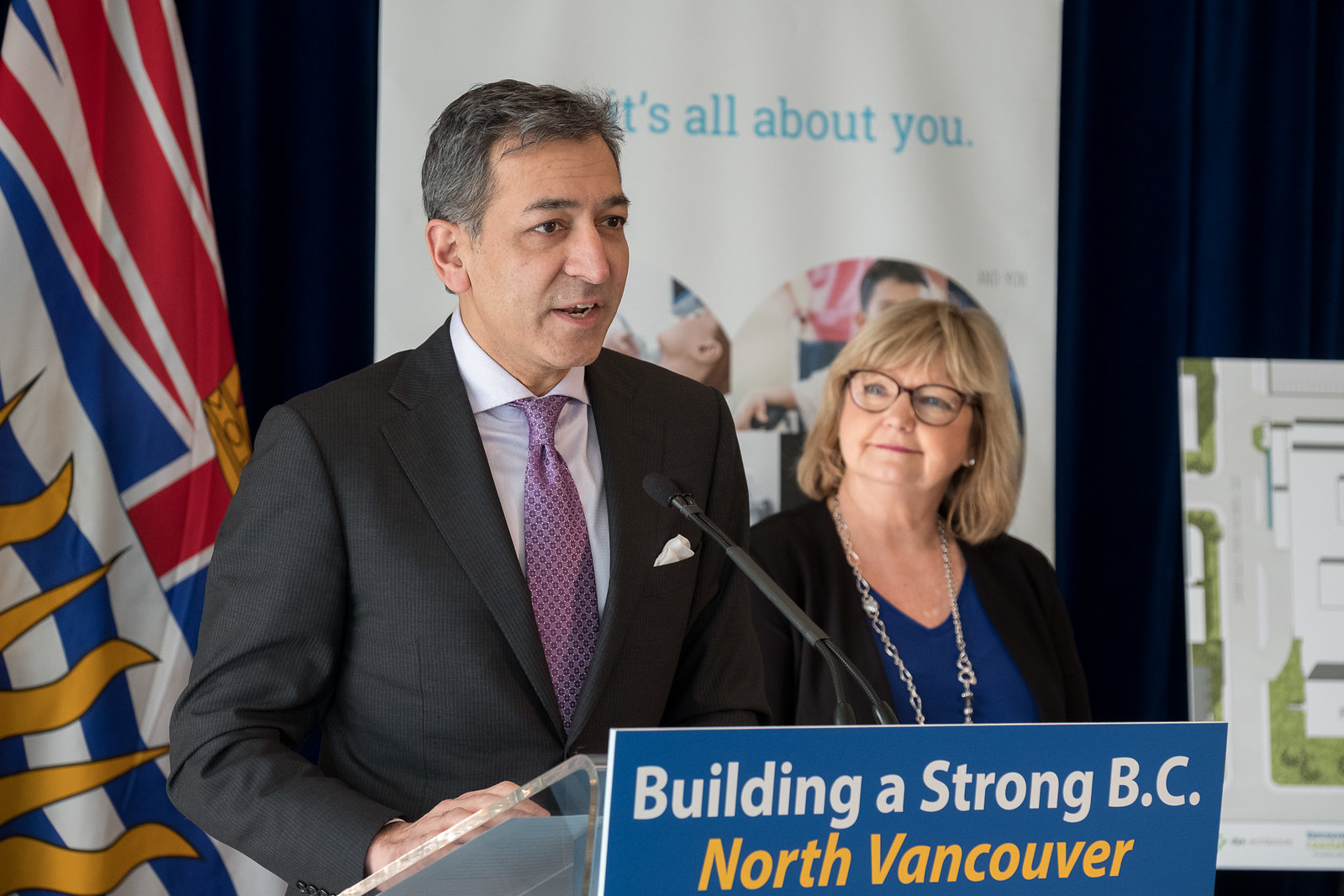In this indoor photograph, a man stands behind a blue podium adorned with text that reads, in bold white letters, "Building a Strong BC," followed by "North Vancouver" in yellow. The man, who appears to be a politician or business leader, is speaking into a microphone attached to the podium. He is middle-aged with black hair streaked with gray and is dressed in formal business attire, including a black suit, a white shirt, and a purple tie.

To his right stands a woman, looking attentively at him. She is wearing a blue blouse, a black jacket, a silver chain necklace, and bold eyeglasses. Behind them, a blue curtain serves as the backdrop, with a flag positioned to the left. Additionally, a large white poster with partially visible text that reads "It's all about you" is also present, adding to the stage setting. The overall ambiance suggests a formal event or speech, emphasizing community and regional development.